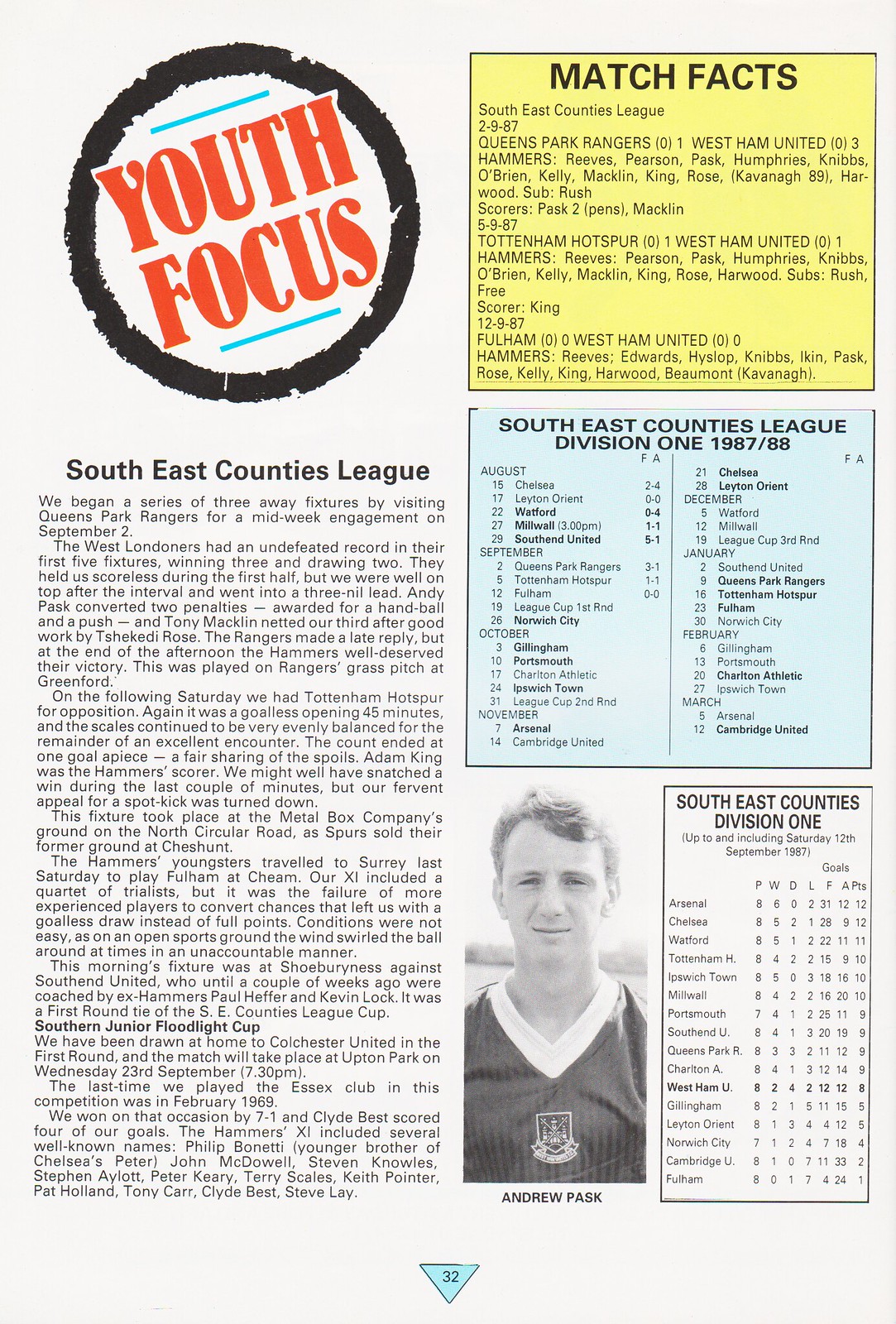The image depicts a page from a sports program or school newsletter, specifically from the sports section. The top left features a black-bordered circle with the words "Youth Focus." Adjacent to this, under the heading "Southeast Counties League," are several paragraphs detailing league information. On the left side of the page, there are standings and historical data for the Southeast Counties League Division One, covering the years 1970, 1987, and 1988.

The right side of the page is divided into three sections. The first section has a yellow background titled "Match Facts," providing specific game-related statistics and player information. Below this, a blue section labeled "Southeast Counties League Division One 1987-88" outlines the league's schedule and standings by month. Prominently featured in the lower right section is a black-and-white photo of Andrew Pask, who is likely a key player instrumental in the league's success. He appears in a football jersey, looking solemnly at the camera, with "Southeast Counties Division One" mentioned again next to his image. The page number, 32, is displayed at the bottom within an upside-down triangle.